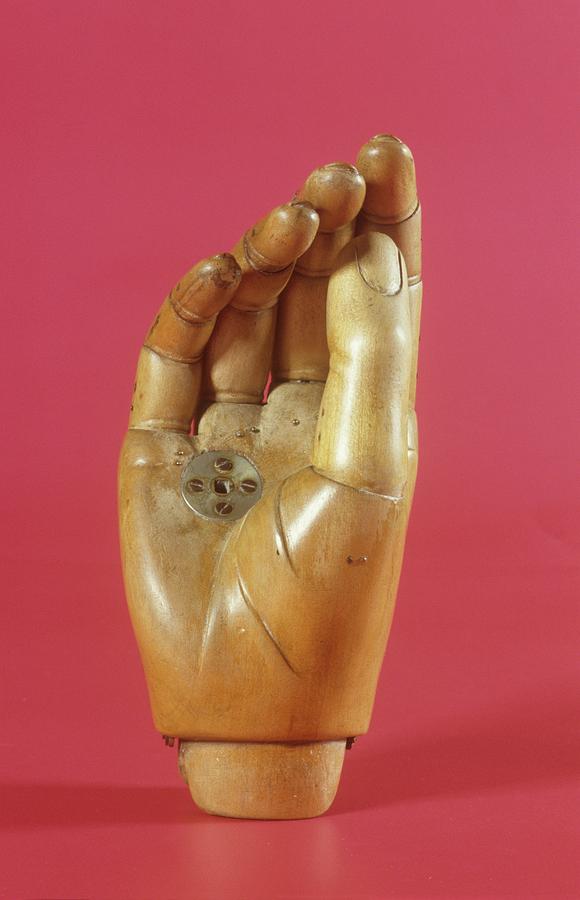The photograph features a detailed, antique wooden model hand set against a reddish-pink background. The right hand, displaying a worn, tan finish indicative of its age, has its fingers bent inward with the index finger positioned highest, descending slightly in height towards the pinky. Central to the palm is a metal disc featuring four screw holes and a central indentation, suggesting it may have previously secured another object. The hand appears purposefully arranged, likely for an auction or magazine, emphasizing its artistic and vintage qualities. Notably, the piece does not extend to a full wrist, instead ending with an attachment piece at the base that supports the hand upright.